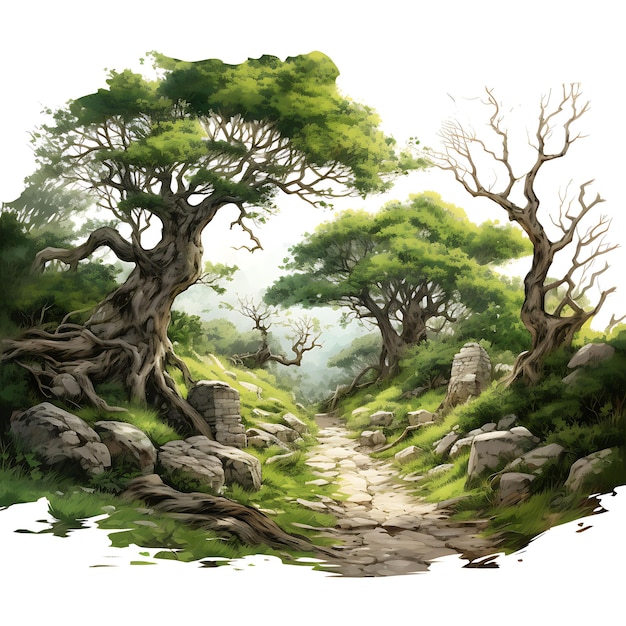The artwork depicts a serene outdoor scene with a narrow, dirt pathway meandering through a picturesque landscape. On either side of the path are grassy hills adorned with large rocks and boulders, some bigger than others. The hillsides feature a mix of trees, including lush green ones whose roots twist and turn visibly above the ground and intertwine with the stones. Among these vibrant trees stand two distinct, bare and twisty trees without leaves, one on each side of the pathway. The scene is enriched with stone block pavers placed on each side for a sturdy walk, emphasizing the natural yet somewhat structured environment. The square-shaped artwork, possibly a painting or digitally generated image, offers no definitive background or border, focusing solely on the tranquil and detailed woodland path that invites the viewer forward into this calm, nature-filled setting on what appears to be a pleasant day.